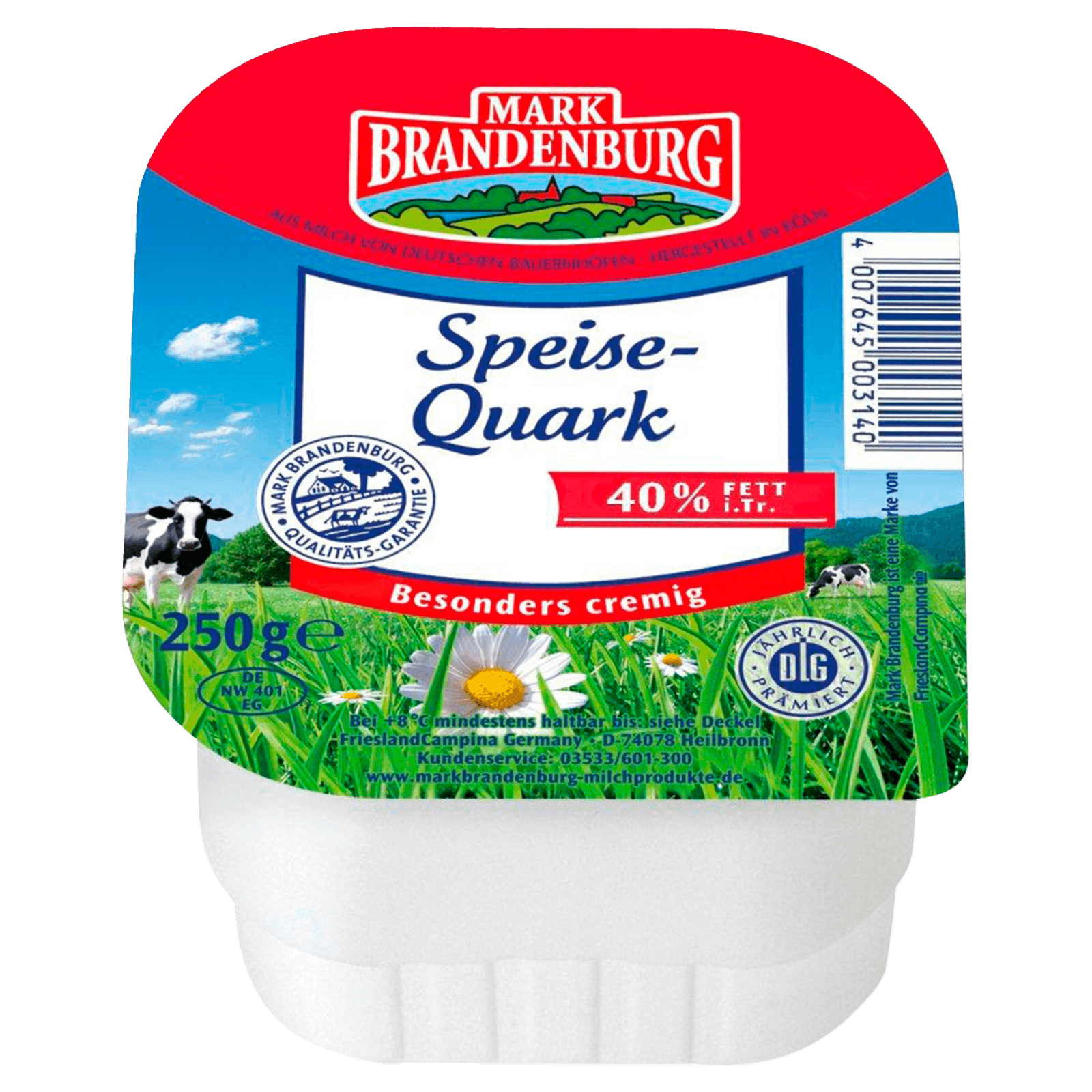The image showcases a highly detailed close-up view of a single object—a container of quark cheese, occupying almost the entire frame against a plain white background. The container is distinguished by its bright, colorful label which is square with rounded corners. The top section of the label is bright red, housing a white-logoed text that reads "Mark Brandenburg," with a green, cartoon-like illustration of a valley below it. The label prominently features a picturesque scene of black and white cows grazing in a lush green field under a blue, cloudy sky. In the foreground, there are clusters of white daisies and green grass. Centered on this pastoral background is another white square containing more text. The text reads "Speise-quark," followed by "40% Fett i.TR." Additionally, there is another "Mark Brandenburg" logo and a red banner with the white writing "Besonders cremig." The label also states that the quark cheese weighs 250 grams. On the left side of the container is a barcode, and there is another circular logo near the center with the text "Jährlich prämiert" wrapped around it. The overall impression is that of a vividly colorful, carefully designed product likely intended for retail display, similar to what one might find in a supermarket listing.